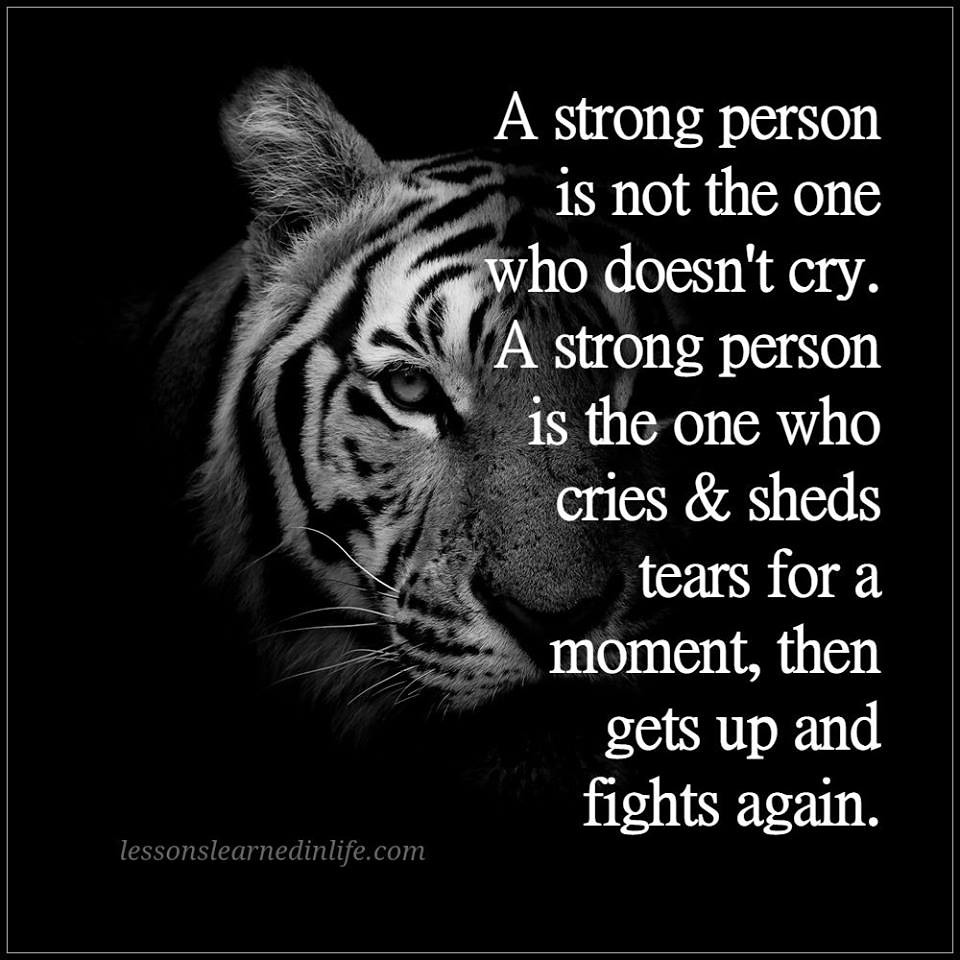In this black and white motivational image, a striking tiger with a partially obscured face commands attention. The tiger's visible half displays intricate stripes, a fuzzy ear, long white whiskers, a dark, imposing nose, and a pair of intense, beautiful eyes. Superimposed on the darkened portion of the image are the words: "A strong person is not the one who doesn't cry. A strong person is the one who cries and sheds tears for a moment, then gets up and fights again." This inspiring message is printed in white lettering. Beneath the tiger's face, in the bottom left corner, the website "lessonslearnedinlife.com" is subtly featured. Encircling the image is a very thin white border, adding a crisp finish to the powerful visual.